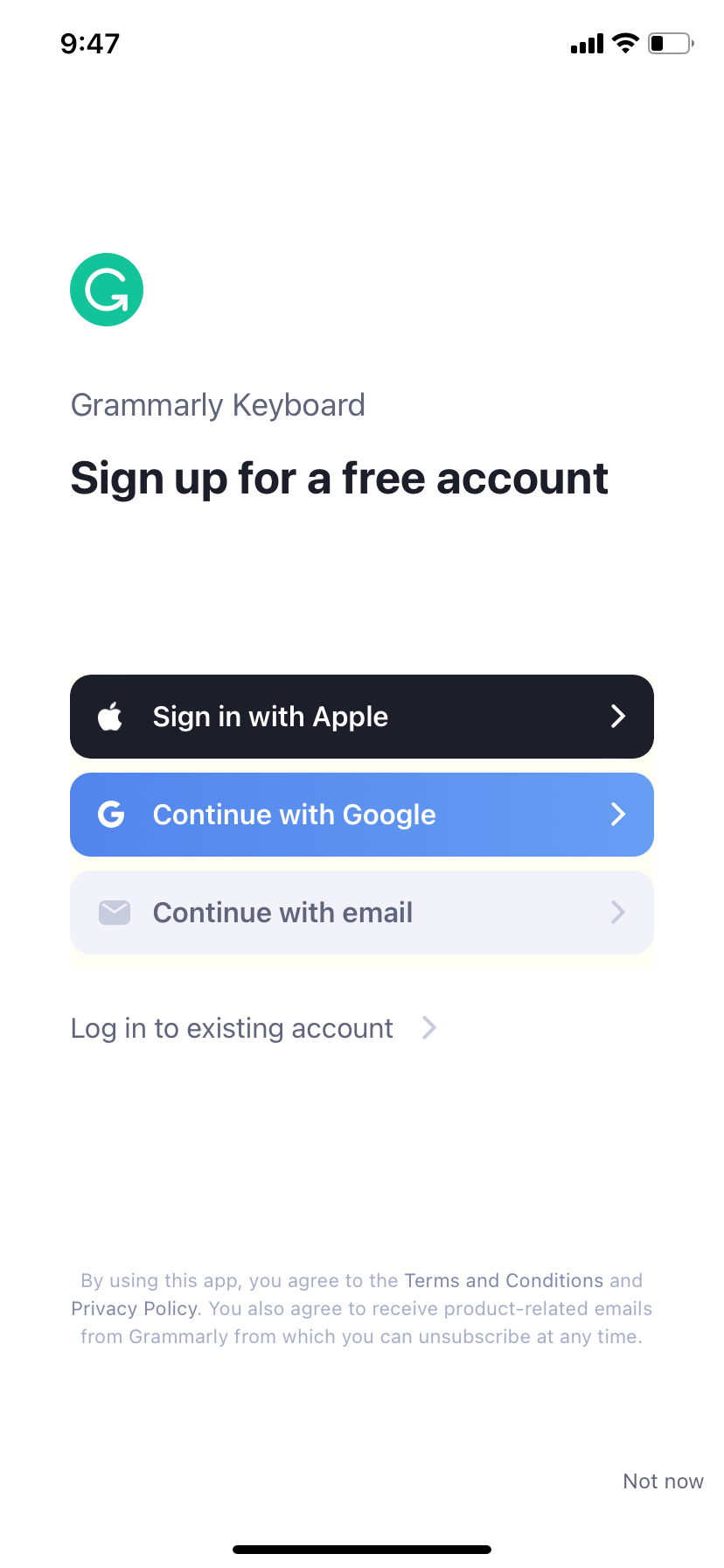A mobile screenshot displaying the sign-in screen for the Grammarly Keyboard app. The top status bar indicates it is 9:47 AM, with full signal strength, Wi-Fi connected, and approximately one-third battery remaining. The screen features a clean white background with black and dark gray text. 

At the center of the screen is the recognizable green Grammarly logo, characterized by a circular arrow shaping a 'G'. Below the logo, the text reads "Grammarly Keyboard". 

The user is prompted to "Sign up for a free account" with three buttons available:
1. A black button with white text and the Apple logo, labeled "Sign in with Apple".
2. A blue button with white text and the Google 'G' logo, labeled "Continue with Google".
3. A light gray button with darker gray text and a gray envelope icon, labeled "Continue with email".

Below these buttons is a link that says "Log into existing account". 

At the bottom of the screen are terms of service details: "By using this app, you agree to the Terms and Conditions and Privacy Policy. You agree to receive product-related emails from Grammarly from which you can unsubscribe at any time."

In the bottom right corner, there is a button labeled "Not now".